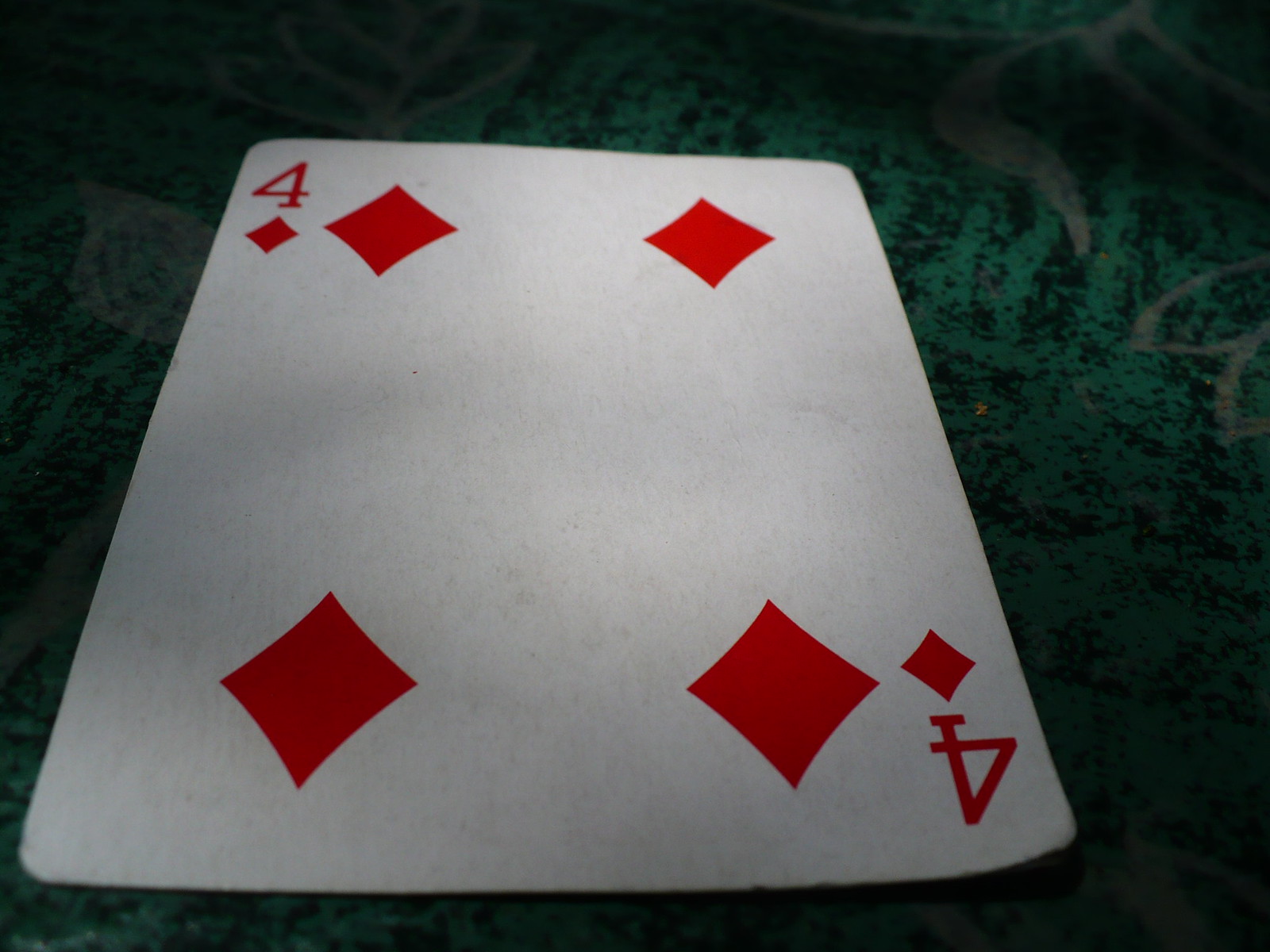The photograph features a single playing card from a deck, set against a dark emerald green background. The background appears to be made of felt, suggesting that the picture was taken on a poker table. The green backdrop is adorned with black dotted prints and intricate grayish filigree designs that become brighter toward the center and darker toward the edges. The playing card, positioned slightly to the left of the frame and captured at a slight angle, displays a red four of diamonds. The card is predominantly white, with a red numeral '4' in both the upper left and bottom right corners, each accompanied by a small red diamond symbol situated just below the numbers. Additionally, the card features four larger red diamond symbols arranged in each corner, slightly set in from the edges. The overall composition creates a visually engaging scene, highlighting the playing card's details against the richly textured background.